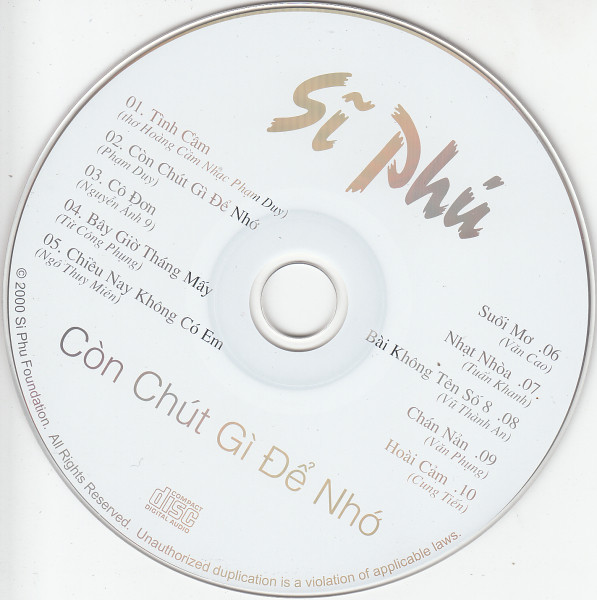This close-up photograph features a CD with a simple, white square background, where the CD itself takes up most of the image. The corners of the square are visible with triangular white cutouts, showing the circular shape of the CD. The cover text appears to be in Vietnamese, prominently displaying "Si Phu" (S-I-P-H-U) diagonally across the center from left to right. The artist's name "Si Phu" and album title "Con Truc Ghi De Ngo" are indicated along with a track list of ten songs, evenly split on the left and right sides of the disc. The first track starts with "01. Tinh Cam," followed by additional text in smaller font, "Tha Hoang Cam Nhac Pham Day" in parentheses, mirroring the format for the other tracks with each having associated text and numbers like "Suoi Mo" and "Van Cao." Along the bottom of the CD, the text reads "Copyright 2000, Si Phu Foundation, All Rights Reserved. Unauthorized duplication is a violation of applicable laws," finished with a Compact Disc logo.